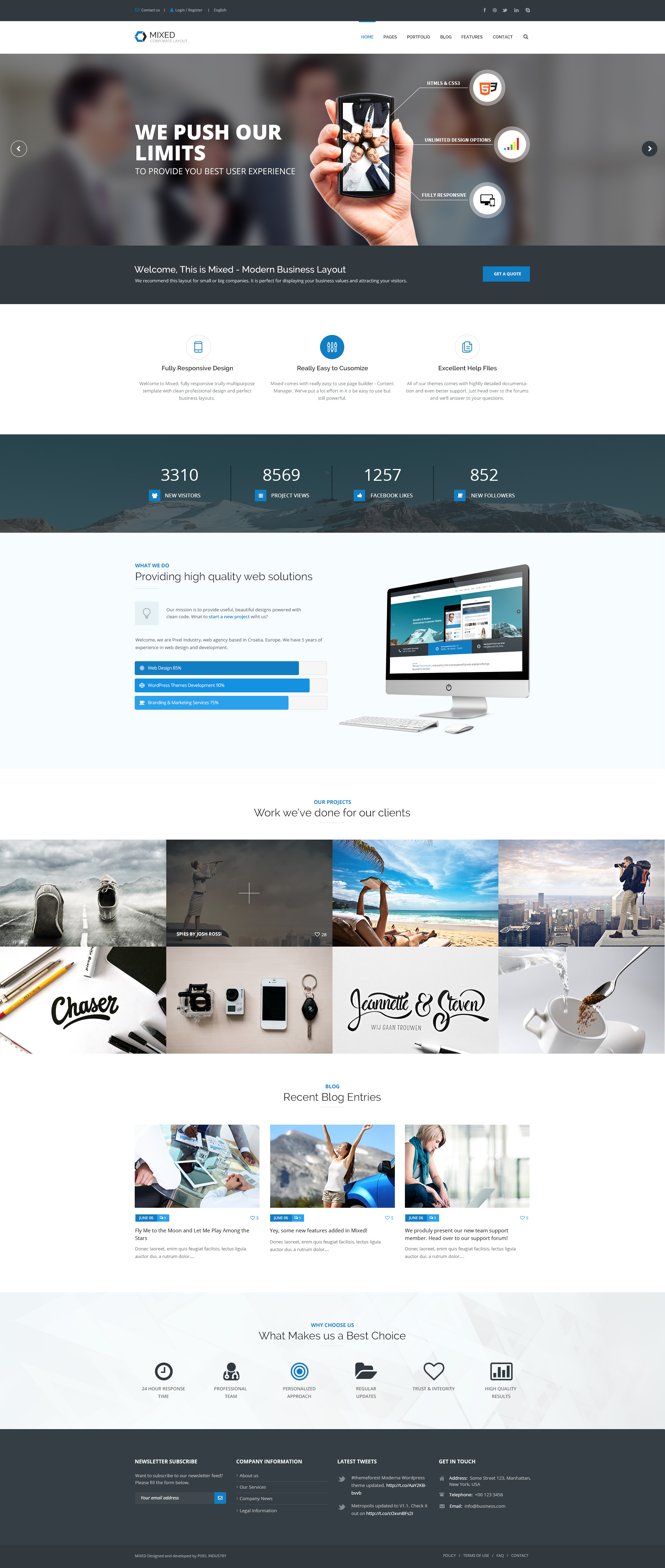The image depicts a webpage that is somewhat difficult to read as it has been made very small in the screenshot. At the top of the page, there is a person holding a cellular phone. Below this, there is a picture showing a group of people standing around, each looking down at their phones. Superimposed in white font are the words "We push our limits." 

From the phone, three bubbles emerge, suggesting wireless connectivity; however, only the first bubble is clearly visible, while the other two are illegible. A blue button with a gray background is also visible on the page.

Additionally, part of the image is blurred out but appears to show two people in business attire, with a woman in the center engaged in a conversation with another woman. A large computer monitor and keyboard are also visible, displaying a blue graphic on the screen. 

Towards the bottom of the webpage, there are several photographs: one featuring a woman with her arms raised in front of a mountain, another showing a coffee cup, and a third capturing a scenic sky with a mountain in the background.